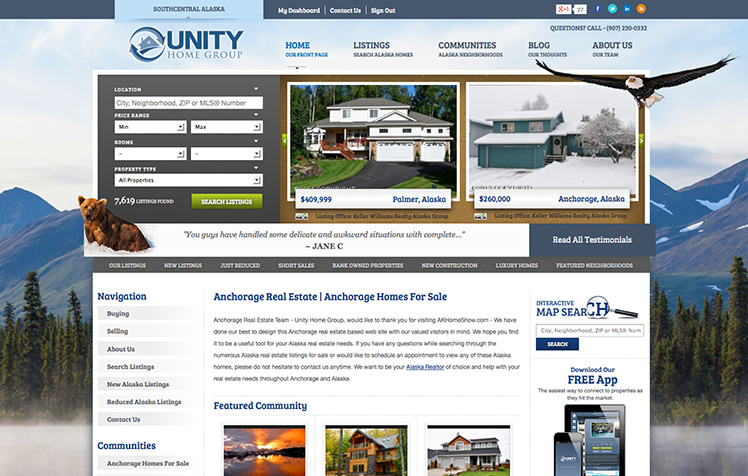The screenshot of the Unity Home Group website prominently features its navigation menu at the top, which includes options like 'My Dashboard,' 'Contact Us,' 'Sign Out,' 'Home,' 'Listings,' 'Communities,' 'Blog,' and 'About Us.' The 'Home' tab is highlighted in light blue, indicating that it is the current page, while the other tabs are displayed in dark blue. 

The central section of the screen contains text and information against the background of a stunning Alaskan landscape. This backdrop showcases picturesque hills, towering mountains, dense forests, and an eagle soaring with outstretched wings, although the eagle appears to be somewhat artificially inserted, detracting from the professional look of the site.

Towards the center of the page, there is a search bar where users can input their desired location, budget, number of rooms, and other preferences. Below this, the website highlights two featured properties with small boxes showing homes in Palmer, Alaska, and Anchorage, Alaska.

Further down, the site provides information about Anchorage real estate, including sections titled "Anchorage Real Estate Homes for Sale,” “Anchorage Real Estate Team," and a warm welcoming message from the Unity Home Group thanking visitors for exploring their site. The text also offers further details about the company and its services.